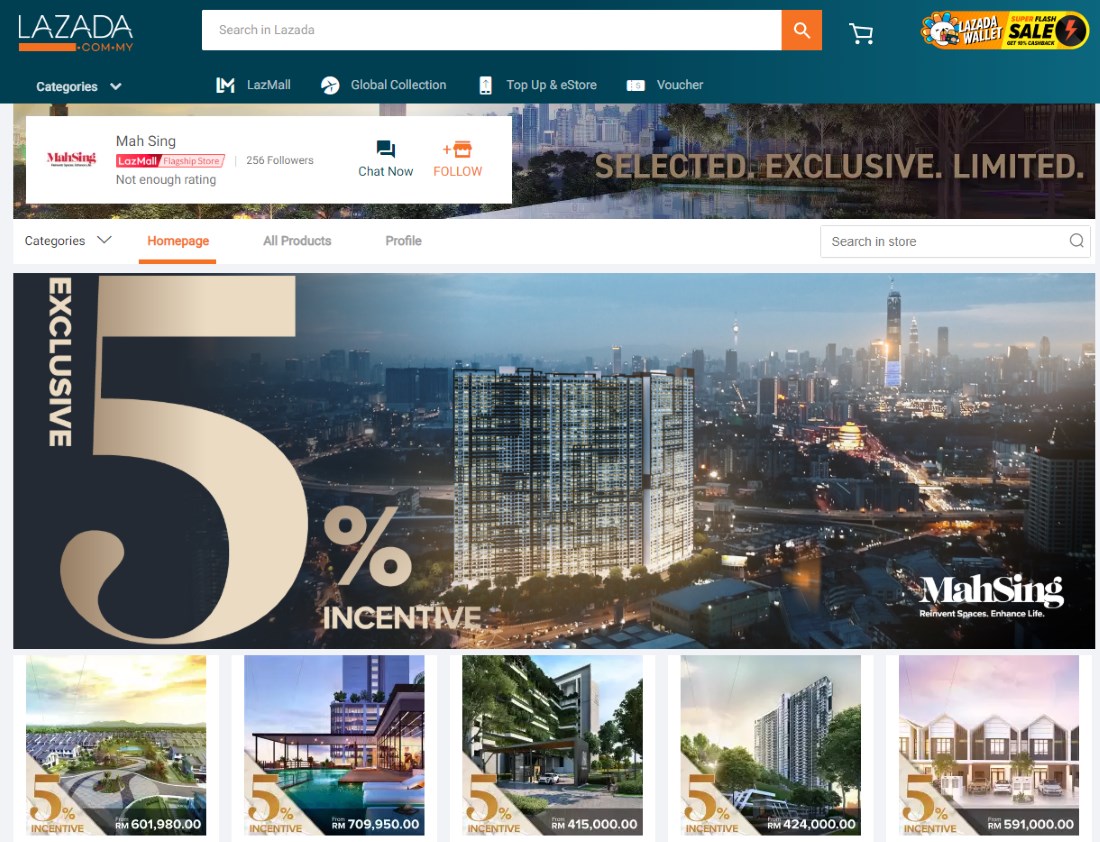The website displayed is Lazada, identifiable by its name "LAZADA" in white, uppercase letters positioned at the top-left corner of the front page. Below the Lazada logo is an orange bar featuring the text "COM-MY" in capital letters. To the right of this bar is a search bar, followed by icons for iShop and Cart. This section of the interface is set on a bluish bar.

Beneath this, a horizontal menu is present, also on its own bluish bar. This bar showcases a city skyline in the background, with text reading "SELECTED . EXCLUSIVE . LIMITED". Further below, there is a vertical menu with categories such as Home Page, All Products, and Profile. Another visual of a city skyline appears underneath this menu, along with a text mentioning a "5% Incentive".